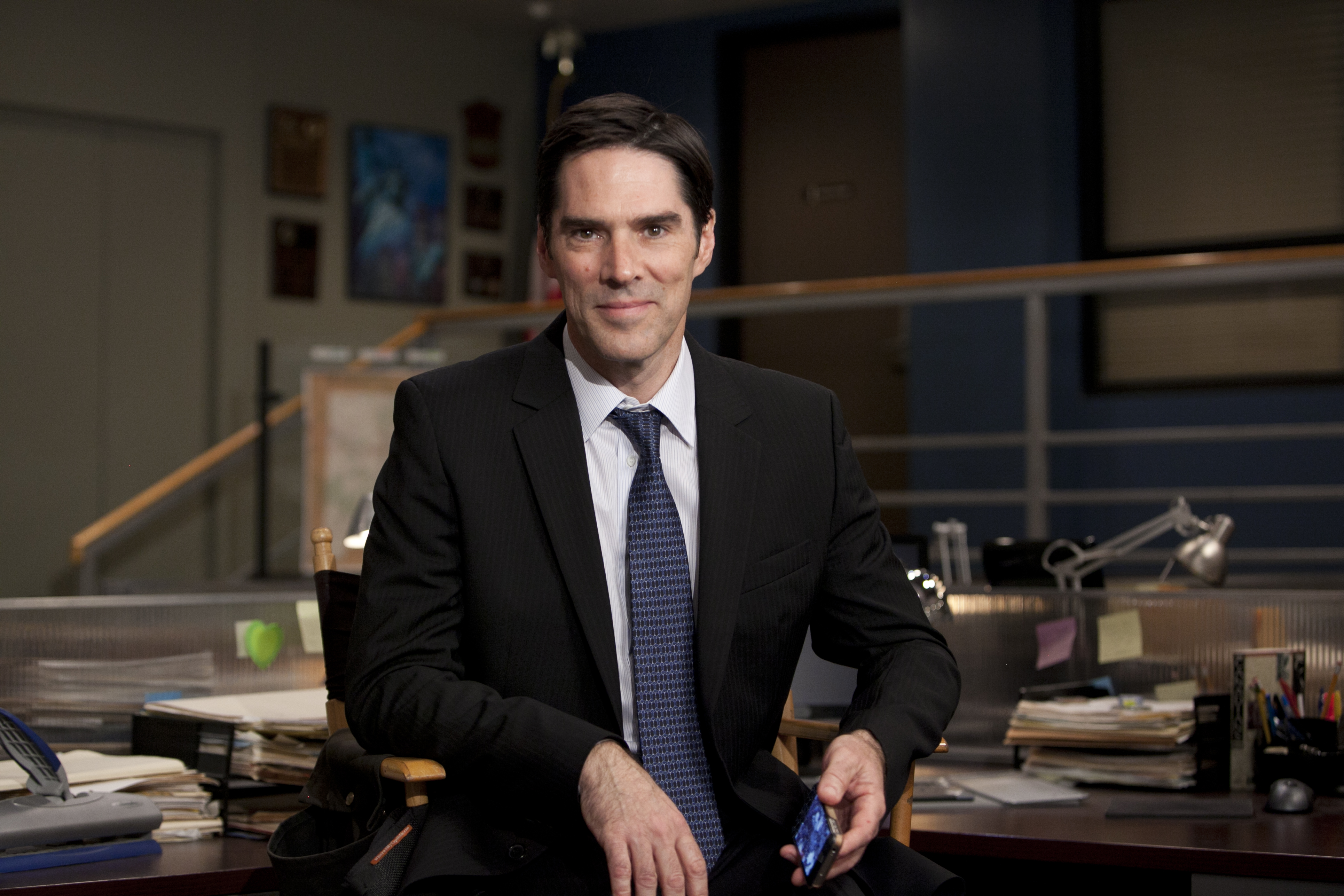This image depicts a man in his late 40s or possibly late 30s, seated in a director's chair, smiling slightly at the camera. He is dressed in a black suit with a white button-down shirt and a blue tie adorned with white dots. The man has short dark brown hair parted to the side and a clean-cut face with a bit of stubble. In his left hand, he holds a cell phone that appears to be on, featuring black accents and possibly silver or gold edges. The setting suggests he is in an office environment, possibly from the show "Criminal Minds." Behind him, the desk is cluttered with numerous stacks of white and yellow papers, folders, sticky tabs in various colors, and writing utensils in black holders. There's a movable silver desk lamp and a pencil holder. The backdrop includes a gray wall, a large window, a brown door with a railing attached to stairs, and additional miscellaneous items hanging on the wall.